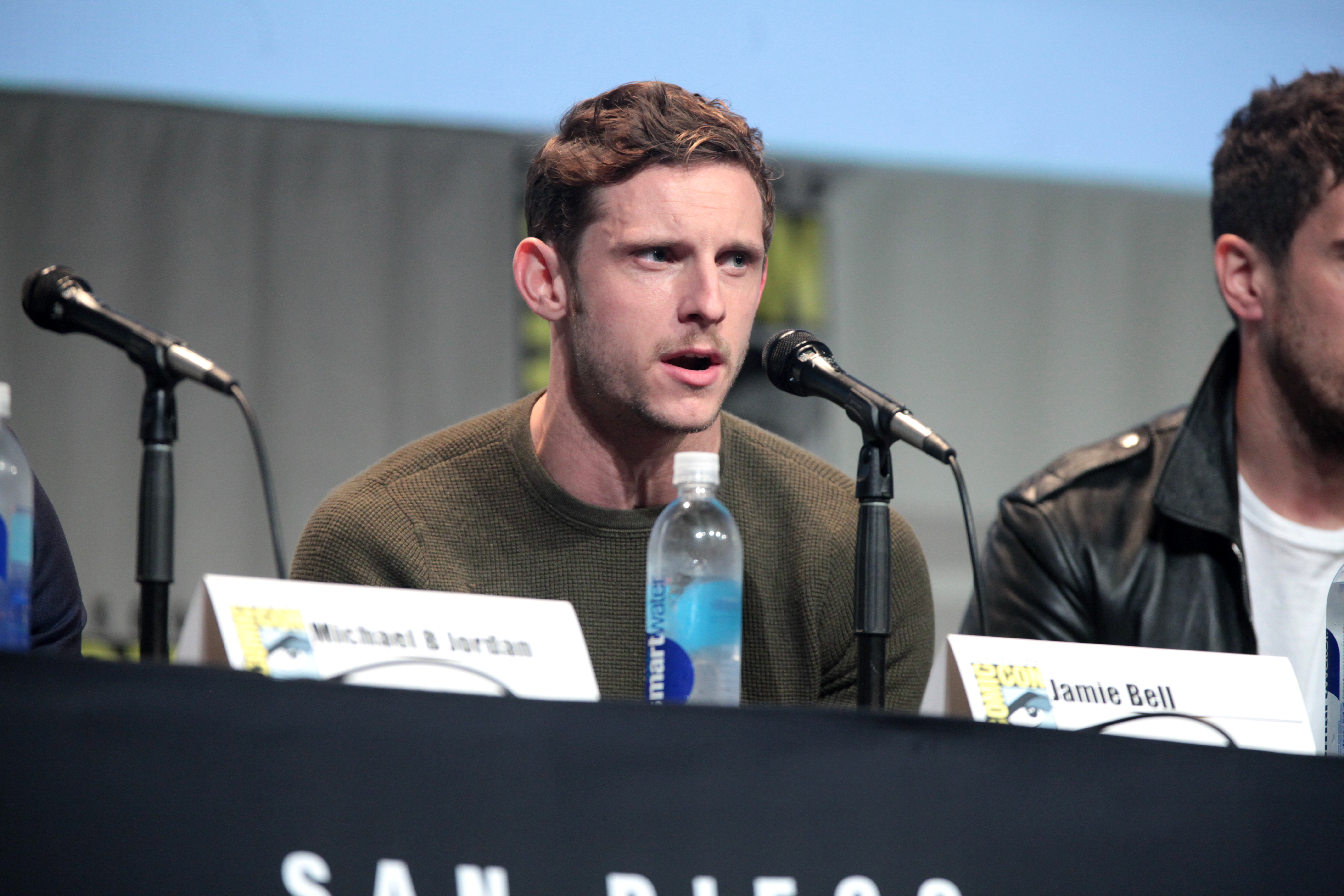The image depicts three men seated at a long table draped with a black skirt, which appears to have partial white lettering suggesting it says "San Diego." The focal point is a man in the center, likely in his late 20s to early 30s, with short brown hair and sideburns, sporting a green sweater. His hands are crossed on the table, and his mouth is slightly open as he looks off to his left, seated in front of a microphone. A bottle of Smart Water is also positioned in front of him, alongside a name card reading "Jamie Bell." To his left, partially visible, is a gentleman in a white t-shirt and black leather jacket. To his right, only a part of the person's arm is visible, suggesting another participant in the scene. The setting seems to be an interview or panel discussion, possibly involving actors or soccer players.